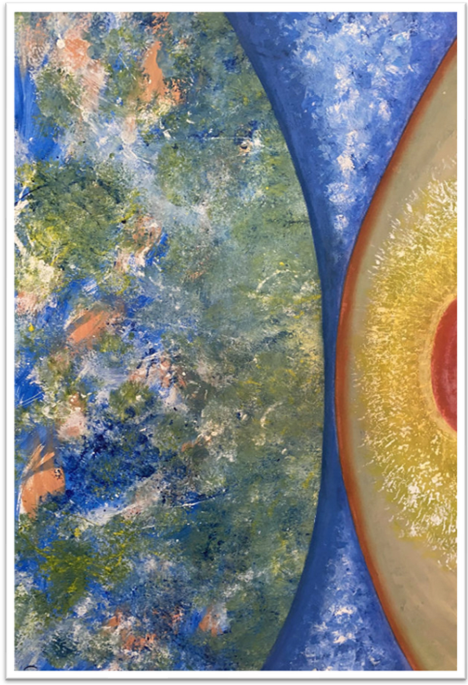The image is a vertically aligned rectangular picture with a white border framing a textured, paint-splattered artistic scene. Dominating the left side and extending slightly past the center is a half-circle with a curved line that arches from bottom to top, filled with various shades of green and blue, accented by touches of brown, yellow, and pastel orange. On the right side, a partial circle in goldish-orange and brown also arches from top to bottom, with a hint of red at its core and orange along its upper edge. Between these two half circles, the area is shaded blue with white, reminiscent of clouds against a clear sky. The overall effect is that of a vivid, multi-colored painting.